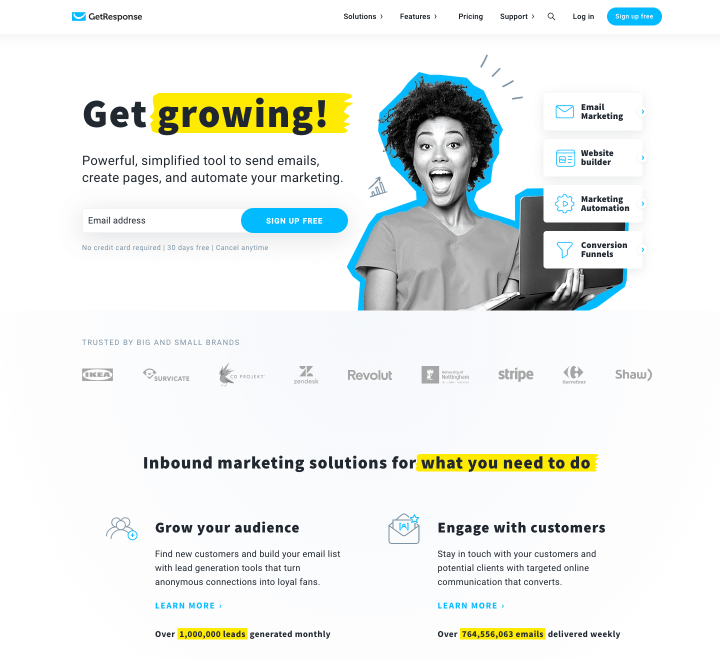A woman is holding a laptop in her hand, prominently displaying a message that reads, "Trusted by big and small brands: IKEA, Cervicats, Revolut, Stripe, Shaw." Below this text, a yellow box highlights the phrase "What you need to do." This is followed by actionable steps: "Grow your audience, find new customers, and build your email list with lead generation tools that turn anonymous connections into loyal fans. Learn more." Additional information notes that over 1 million leads are generated monthly. The caption continues, "Engage with customers. Stay in touch with your customers and potential clients with targeted online communication that converts. Learn more." An impressive statistic concludes the message: "Over 764,556,063 emails delivered weekly."